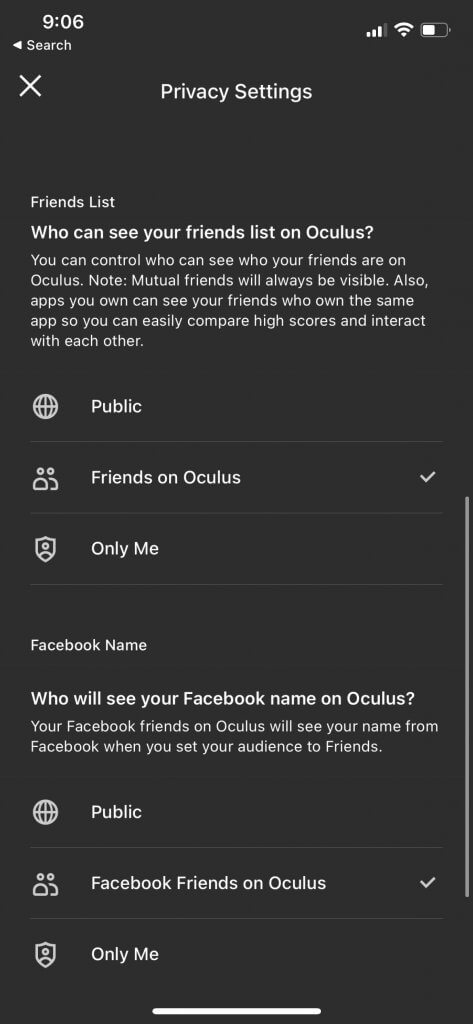**Detailed Caption:**

This image displays the privacy settings for the Oculus VR platform, captured at 9:06. The top of the screen clearly indicates the option to manage 'Friend List' settings. This section allows users to control who can view their friends list on Oculus. Users can customize their settings so that mutual friends are always visible. Additionally, applications can access the friends list to show which friends own the same app, facilitating easy high score comparisons and interactions within the app.

The settings also specify how public information is managed, particularly in relation to Facebook. Friends on Oculus will see the user's chosen name, whereas public Facebook friends list settings ensure that only specific information is visible. When sending friend requests, the name associated with the user's Facebook account will be shown to others.